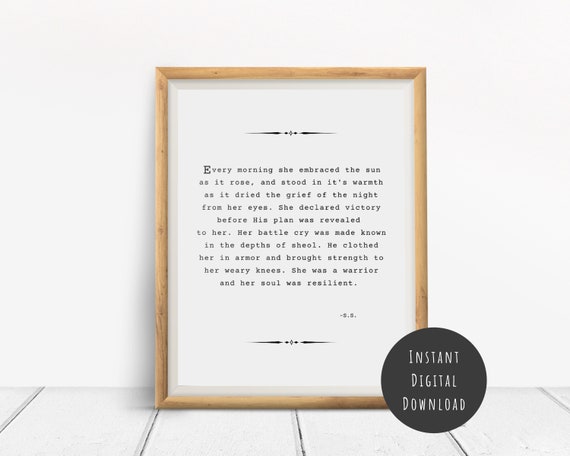The image depicts a piece of framed text against a plain white wall, resting on a surface of white painted wood. The frame is crafted from light brown wood. In the lower right corner of the image, there is a dark gray circle with the phrase "Instant Digital Download" written in white text, indicating the nature of the product. Within the frame, there are elegant dividers at the top and bottom, and the text reads: "Every morning she embraced the sun as it rose and stood in its warmth as it dried the grief of the night from her eyes. She declared victory before his plan was revealed to her. Her battle cry was made known in the depths of Sheol. He clothed her in armor and brought strength to her weary knees. She was a warrior and her soul was resilient." While there are initials at the end of the quote to attribute it, they are too small to decipher. The image appears to be an advertisement for a digital product available for download, allowing customers to print and frame the quote themselves.